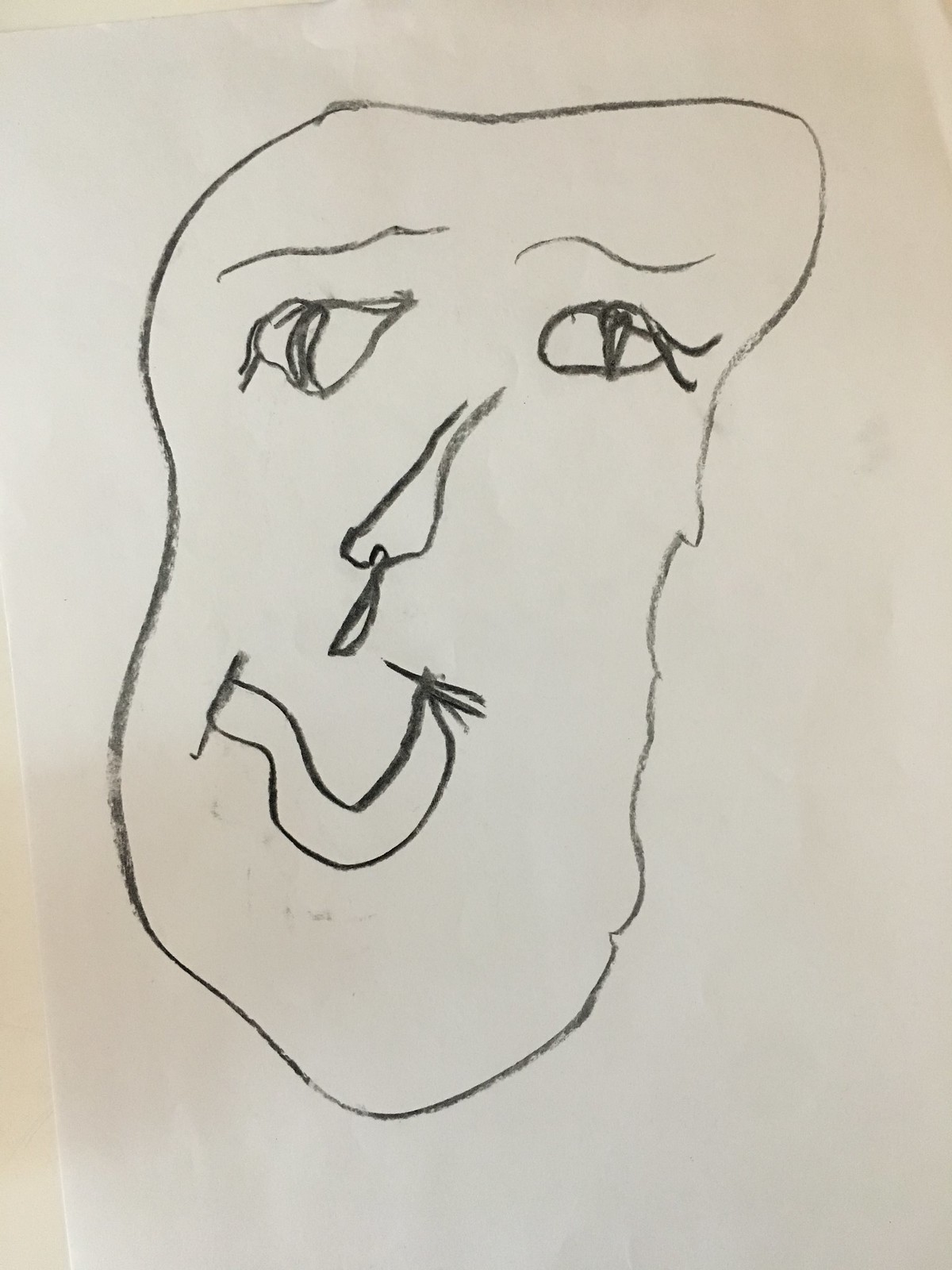This photo captures a crude pencil drawing of a face, likely created by a child, on an off-white, slightly wrinkled piece of paper. The face has a rough, potato-like shape with jagged edges, making it asymmetrical and warbled at both the top and bottom. The eyes are differently shaped, each with vertical, scribbled-in pupils and attempts at eyelashes. The eyebrows are simple, curly lines positioned above the eyes. The nose, resembling a loop with an extra line at the bottom, creates the impression of something hanging from it, possibly snot. The mouth is drawn as a warbled U shape with two lines, indicating an open smile, and has additional lines at the sides to represent smile lines. The drawing lacks details such as ears, hair, and a neck, enhancing its crude and childlike appearance. The background surface is also off-white, visible at the bottom left corner where the paper edge lifts slightly.